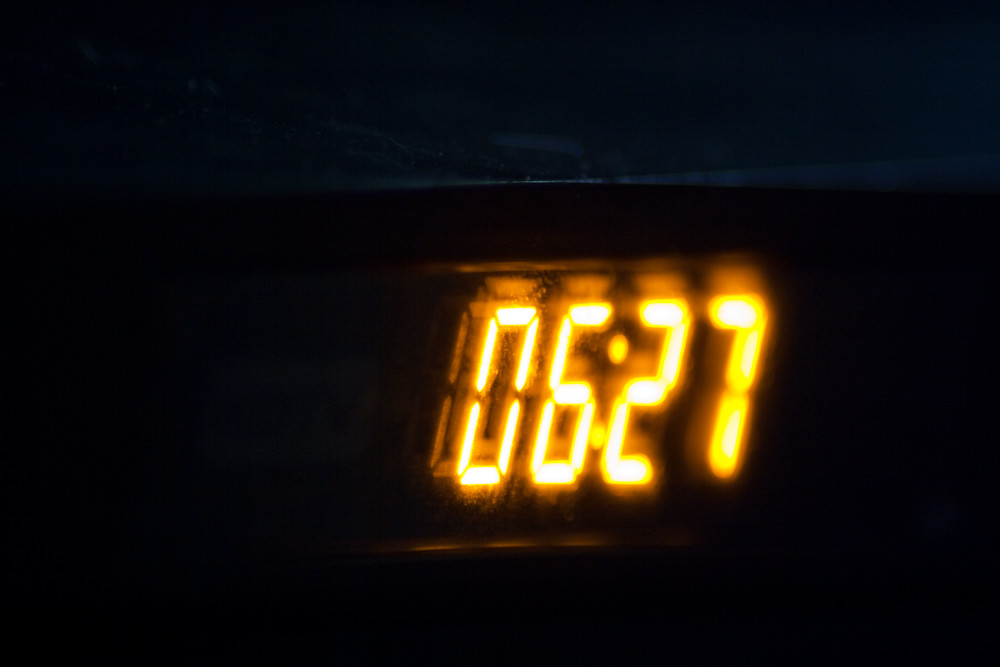This photograph captures a digital alarm clock prominently centered in an otherwise completely dark scene. The background and the clock itself are both pitch black, suggesting the picture was taken at night with no external light sources. The only illumination comes from the clock’s glowing LCD display, which shows the numbers 0627 in a bright amber hue, almost resembling a fire-like glow. These yellowish-orange digits not only stand out due to their vibrant color but also cast a slight reflection above and below them, emphasizing their luminosity in the darkness. The numbers are likely indicating the time as 6:27 AM. Despite the starkness and minimalism of the image, the vivid digital display draws all the attention, creating a captivating contrast against the deep black surroundings.